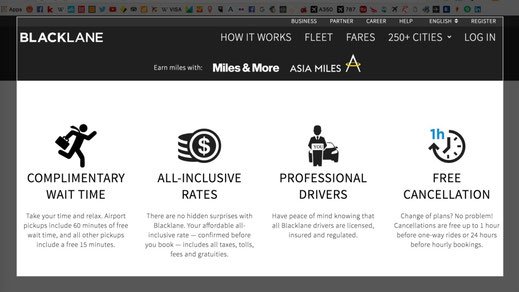This is an image from the company Black Lane, evident from its name printed prominently in white at the top of the website. The top of the webpage also features faint icons in light gray, meant to be navigational tools for the desktop version of the site. Adjacent to the "Black Lane" logo, the menu options read "How It Works," "Fleet," "Fares," "250+ Cities," alongside a dropdown arrow and a "Login" button. Above this main navigation bar, there is an additional black section displaying links for "Business," "Partner," "Career," "Help," "English," and the status "Registered."

Further down on the black section, a footer mentions "Email," and alliances like "Earn Miles with Miles & More" and "Asia Miles," ending with a large tan "A". 

Below this, a large white section details the company's offerings: 
- "Complimentary Wait Time": Customers can take their time and relax, as airport pickups include 60 minutes of free wait time, while other pickups offer 15 minutes of free wait time. This section is illustrated with an icon of a running man. 
- "All-Inclusive Rates": Promises no hidden surprises as all-inclusive rates are confirmed before booking and cover taxes, tolls, fees, and gratuities. Represented by a dollar sign icon.
- "Professional Drivers": Assures peace of mind, stating that all Black Lane drivers are licensed, insured, and regulated, accompanied by an icon showing a driver with a sign in front of a car.
- "Free Cancellation": Offers flexibility, as cancellations are free up to one hour before a one-way ride or up to 24 hours for other bookings. This information is depicted with an icon of a clock indicating one hour in blue.